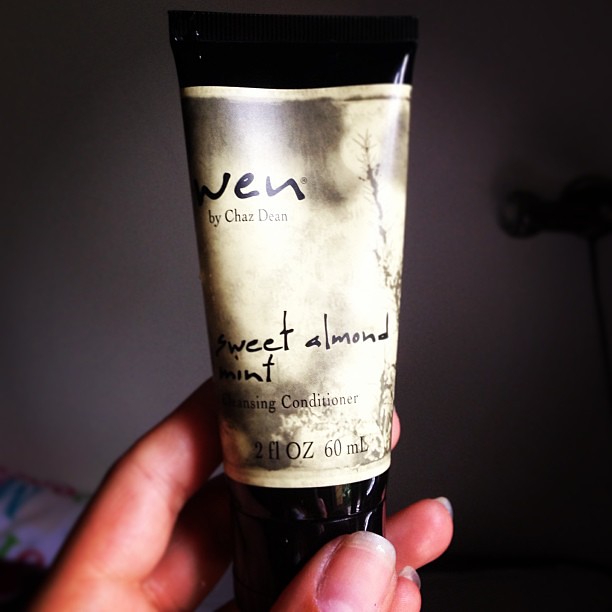This color photograph, taken in an indoor setting, showcases a tube of hair care conditioner prominently displayed against a dark gradient background. The subject of the image is held by a hand with fingers wrapped around the base of the tube, and the square format allows for a detailed view of the product. The tube features a black top and bottom, with a cream-colored middle section adorned with text and a blurred landscape design. The text on the tube includes phrases such as "When by Justine," "Sweet Almond Mint Cleansing Conditioner," and "2FL-OZ 60 ml" written in black letters. Despite the darkness of the room, which casts uncertainty on the exact color of the background wall, possibly pink, the overall style adheres to photographic realism with a focus on product representation. The tube appears to be turned upside down, as if to dispense the last of its contents, presenting a practical and realistic depiction of the product's use.